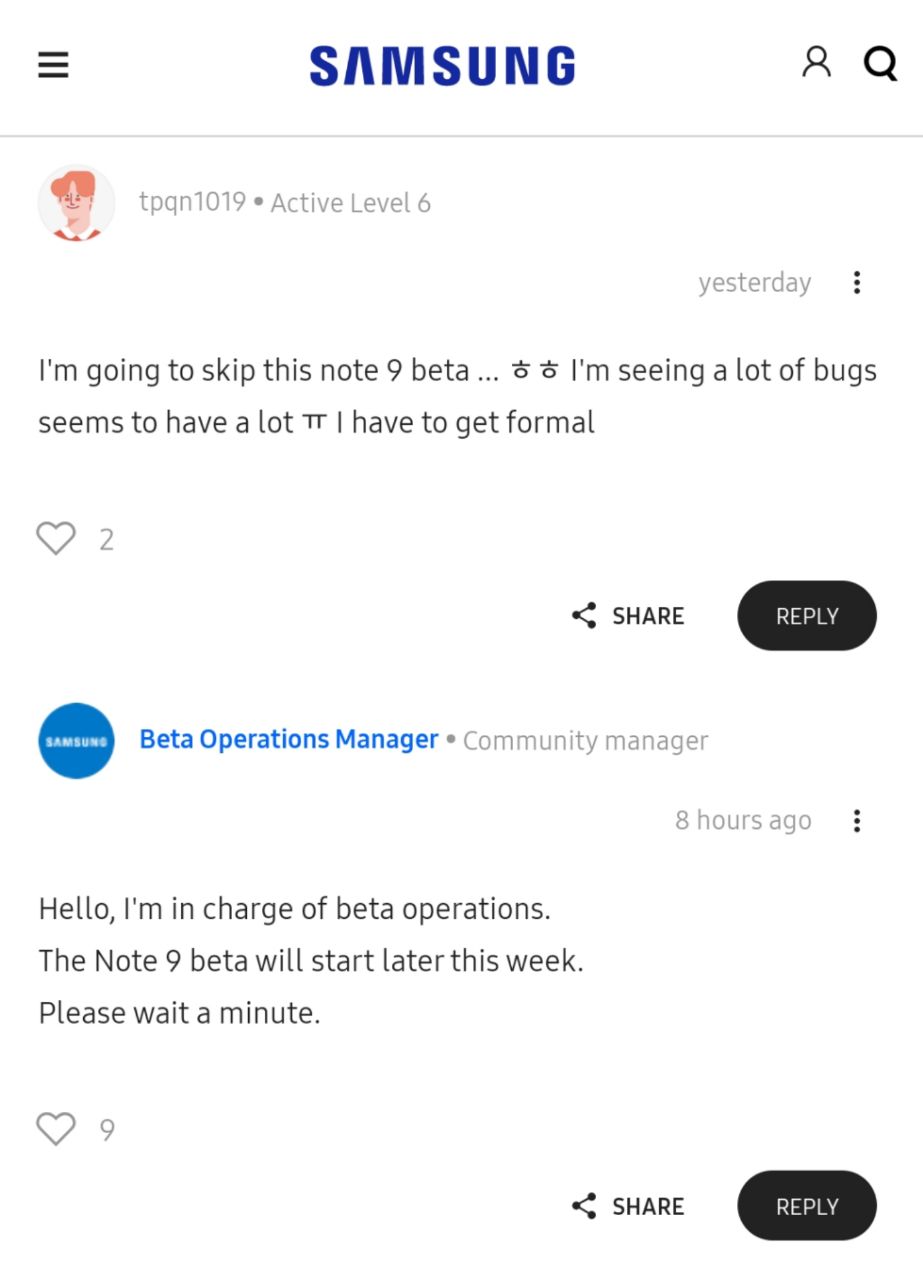This is a detailed screenshot of a conversation between a user and Samsung, showcased in a clean and structured format. At the top of the screenshot is a menu icon represented by three horizontal lines, followed by the name "Samsung" in bold blue letters at the center. On the right side of the header, there is a user ID icon and a search icon. Below this header is a thin gray line demarcating the section.

Immediately beneath the gray line is a circular user avatar, which is a cartoon image depicting a user with orange hair, wearing a white top with orange accents. Next to the avatar is the username "TPQN1019," marked with a circle indicating an active level six status. The timestamp shows the message was sent "yesterday." 

The message from the user reads: "I'm going to skip this Note 9 beta... I'm seeing a lot of bugs, seems to have a lot, pie, I have to get formal." This message has garnered two likes, as indicated by a heart icon with the number "2" beside it. Underneath the message, there are share and reply icons; the reply button has a black background with white text.

Samsung's response is highlighted below this section. A blue circle with the word "Samsung" marks the start of the reply, accompanied by the username "Beta Operations Manager, Circle Community Manager." Samsung's response was posted eight hours ago and reads: "Hello, I'm in charge of beta operations. The Note 9 beta will start later this week. Please wait." This reply has received nine likes, denoted by a heart icon with the number "9" beside it.